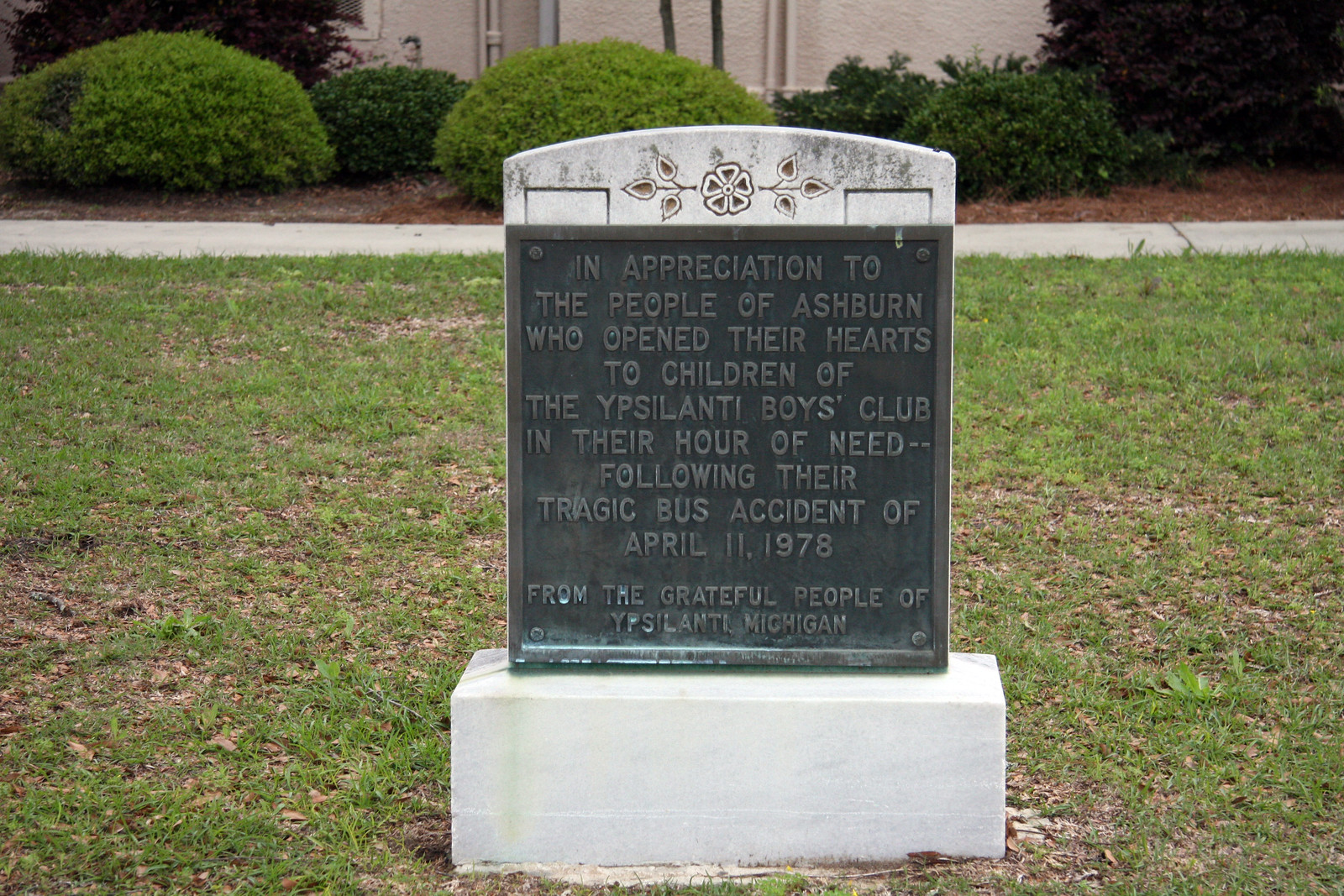This image depicts a memorial sign placed in a grassy area with a sidewalk and several green bushes in the background. The sign stands on a white rectangular pedestal with a dark gray metal plaque mounted on top. The plaque is adorned with intricate designs featuring a flower and vine motif in a dark brown color at the top. The inscription on the plaque reads: "In appreciation to the people of Ashburn who opened their hearts to children of the Ypsilanti Boys Club in their hour of need following their tragic bus accident of April 11th, 1978. From the grateful people of Ypsilanti, Michigan." The memorial is situated on patchy green and beige grass, highlighting its somber yet appreciative message.